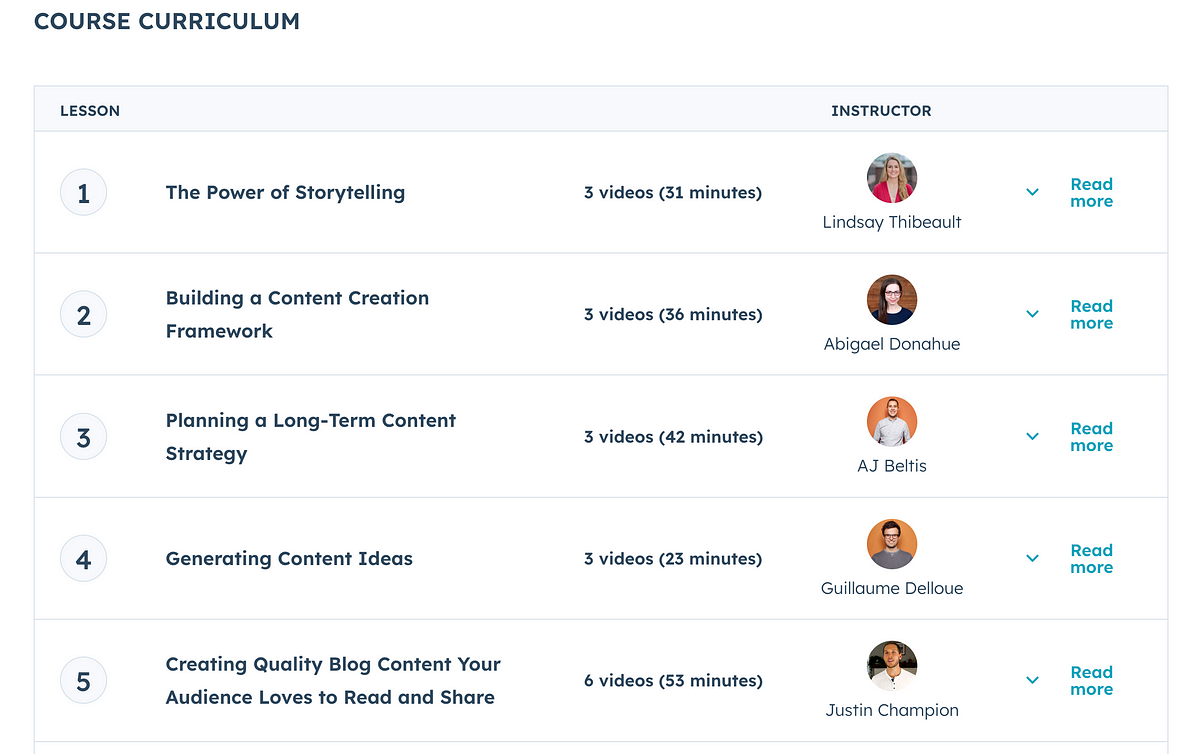The image showcases an online course curriculum detailing the first five lessons. Each lesson includes the instructor's name, description, and video length:

1. **The Power of Storytelling**
   - Featuring three videos totaling 31 minutes.
   - Instructor: Lindsay DeBalt, a Caucasian woman with blonde hair, wearing a red blouse, and standing outside.

2. **Building the Content Creation Framework**
   - Comprising three videos summing up to 36 minutes.
   - Instructor: Abigail Donahue, a Caucasian woman with long black hair, dressed in a black shirt, and positioned against a brown wall.

3. **Planning a Long-Term Content Strategy**
   - Encompassing three videos for a total of 42 minutes.
   - Instructor: AJ Beltis, a Caucasian man with short brown hair, wearing a long-sleeve shirt, and standing in front of a brown or orange wall.

4. **Generating Content Ideas**
   - Containing three videos with a total duration of 23 minutes.
   - Instructor: Gilliam Delahue, who appears preppy with short black hair, glasses, and a gray shirt.

5. **Creating Quality Blog Content Your Audience Loves to Read and Share**
   - Consisting of six videos, adding up to 53 minutes.
   - Instructor: Justin Champion, a young Caucasian man with short hair on the sides, wearing a white shirt.

Each lesson includes a 'read more' button for additional details.